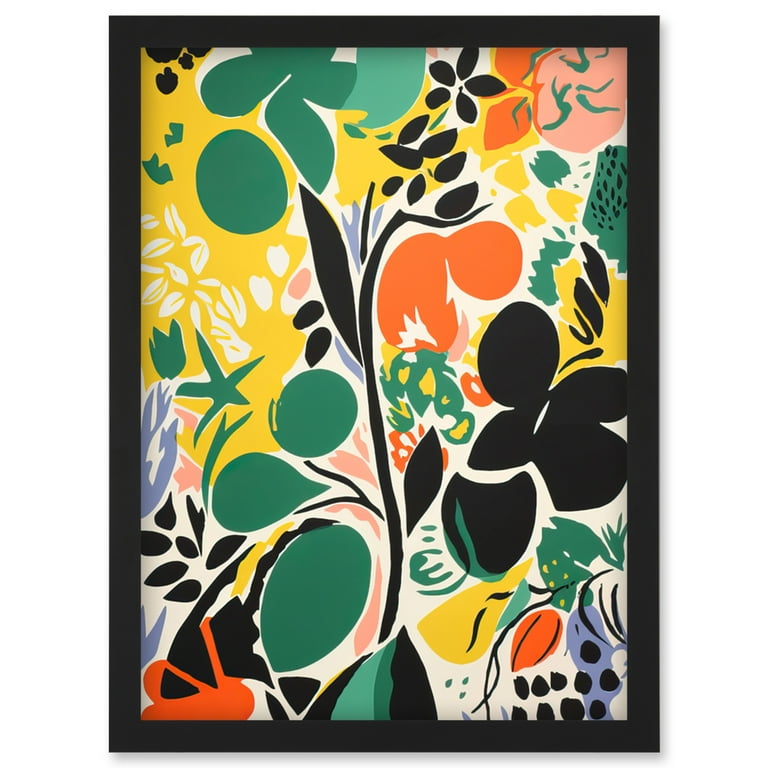This highly stylized and abstract painting is framed in a thin black or nearly black border and hangs on a white wall. Its background is predominantly yellow, accentuated by vivid splashes of colors such as green, red, orange, black, teal, and white. The central focus appears to be a dark, black silhouette of a plant, featuring a stem, leaves, and blooming flowers. Surrounding this are smaller, round elements that resemble leaves or fruits, adding to the impression of vegetation or a nature scene. Throughout each quarter of the painting, abstract shapes in greens, yellows, reds, and blacks are scattered, contributing to its floral and lush composition. Despite its detailed depiction of plant life, the painting maintains an air of abstraction, leaving specific details to the viewer's interpretation. There is no writing or artist's signature visible, and no humans, animals, structures, or mechanical objects are present in the artwork.